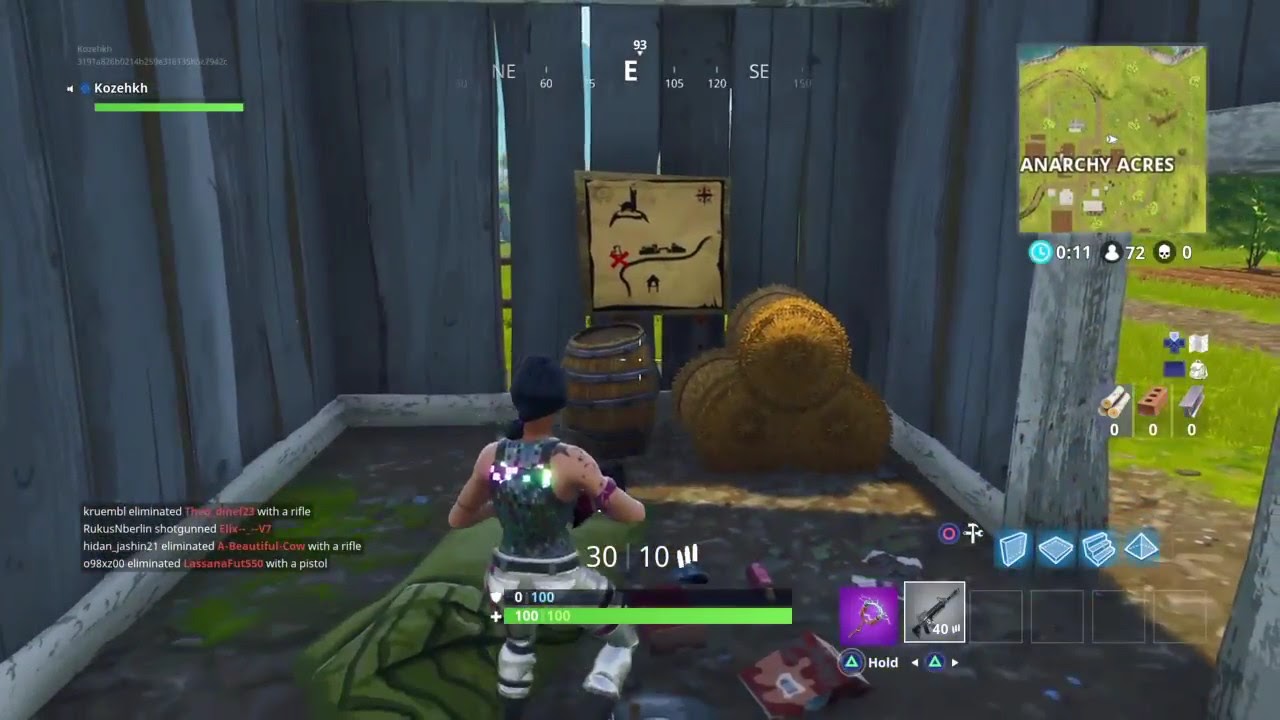This screenshot from a video game captures a rustic interior of a gray, wooden structure with vertically aligned boards and visible cracks between them, revealing green grass and a tree outside. The building, somewhat resembling a shack with gray wooden trim, features a doorway without a door on the right wall. Inside, a person with black hair tied in a ponytail is kneeling on the dirt floor. They are dressed in a darker tank top, which appears sparkly or sequined, and white pants with knee pads and a black belt. An armband adorns their right upper arm. This individual, viewed from the back and facing a far wall, has muscular arms and appears to be looking at an old whiskey keg. Above the keg is a tan map outlined in black, featuring a squiggly road line and a red "X," indicating a significant location.

To the right of this map are three rolled bales of hay standing upright. Scattered around the dirt floor, which includes patches of green moss and rocks, are various items and what might be a green sleeping bag.

On the top-right of the screen is a mini-map indicating "Anarchy Acres" in white letters, and adjacent to it is a time display showing "0:11." There is a silhouette of a person marked with the number 72 and another icon featuring a skull with a "0" next to it. Below this section is a partially visible username, "Kosen K H." More text and numbers appear in the bottom-left corner, mostly in white with some red font, representing user stats or in-game messages. Additionally, a green bar and a longer green power bar reading "100 out of 100" are present. 

The upper-middle section of the screen also contains a compass with directional markers including "E" for East, "NE" for Northeast, and "SE" for Southeast. Next to the figure's back are white numbers, "30" and "10," with a black strip and a green strip showing white numbering below them. Further right are six squares; two contain objects, one being purple and the other gray, possibly indicating weapons, while additional icons are seen above them.